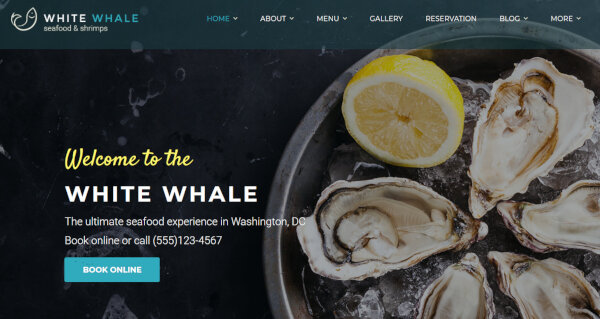The top left of the image features the text "White Whale" with "White" in white font and "Whale" in blue font. Below the name is the word "Seafood" and a representation of shrimps. Adjacent to this on the left side, there's a small icon depicting a fish in white.

On the right side of the image, there is a navigation menu with several options. The "Home" option is highlighted in blue, while the other options—"About," "Menu," "Gallery," "Reservation," "Blog," and "More"—are displayed in white. Some of these options have small, downward-facing arrows next to them, indicating dropdown menus.

Beneath this navigation menu, the text "Welcome to the White Whale" is showcased with "Welcome to the" in yellow and "White Whale" in white. Following that, in smaller text, is a tagline: "The ultimate seafood experience in Washington DC." Instructions for booking are provided: "Book online or call (555) 123-4567," accompanied by a blue button with "Book Online" written in white text.

The background of the image features a metal bowl positioned on the right. Inside the bowl are several clams, a slice of lemon, all resting on a bed of ice, adding a visual representation of the fresh seafood offered by the establishment.